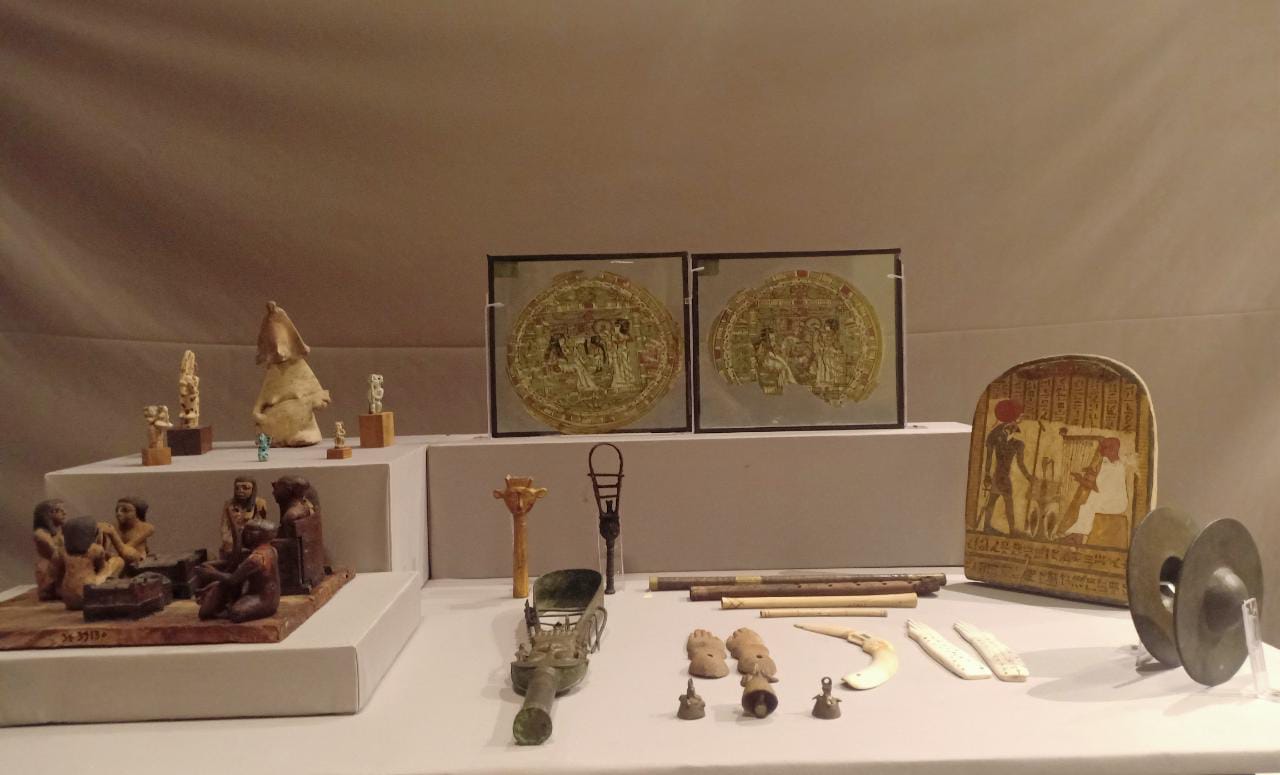The image depicts a detailed museum display featuring a variety of ancient Egyptian artifacts arranged on a white tabletop. Behind the table, a beige sheet serves as the backdrop, enhancing the visual focus on the items. On the table's right side, there is a tablet adorned with Egyptian hieroglyphs and illustrations, including a person playing a harp-like instrument before a pharaoh. Scattered across the table are small metal symbols and wooden wind instruments, resembling flutes, along with other unidentified objects made of metal and wood.

To the left on a higher white platform, there are small wooden carvings representing people. These carvings depict a group of at least six individuals, with one seated in a chair and another playing a string instrument nearby. In the upper left section, additional wooden figurines rest on a brown cutting board-like surface. 

Framed artwork, likely Egyptian in origin, is positioned toward the back of the display. These frames contain pieces of fabric impressed with Egyptian designs, emphasizing the theme of ancient Egyptian music and daily life. Notable among the artifacts are stone carvings and a plaque featuring an illustration of Horus. The overall setup suggests an educational exhibit focused on the musical culture and artifacts of ancient Egypt.